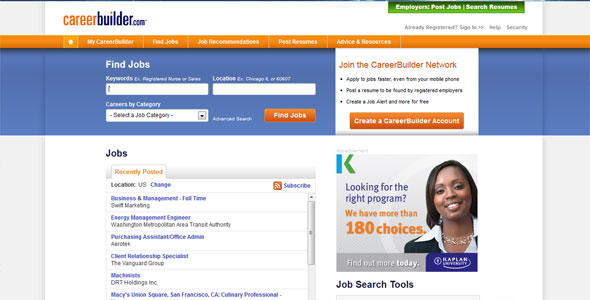This image from CareerBuilder.com showcases a comprehensive job search and career development platform. The webpage features multiple functionalities including options to find jobs, receive job recommendations, post resumes, and access career advice and resources. For registered users, there is a sign-in option. Employers can benefit from features like job postings and resume searches. 

A prominent banner invites users to join the CareerBuilder network, enabling faster job applications, including from mobile devices. Users can post their resumes to be discovered by registered employers and create job alerts for free. The interface includes text fields for entering keywords and job locations. 

The page lists various job openings such as Business and Management Full Time, Energy Management Engineer, Purchasing Assistant, Office Admin, Client Relationship Specialist, Machinist, and Culinary Professional. Specific job locations mentioned include Mrs Union Square in San Francisco, California. The layout is designed to assist both job seekers and employers in accomplishing their respective goals efficiently.